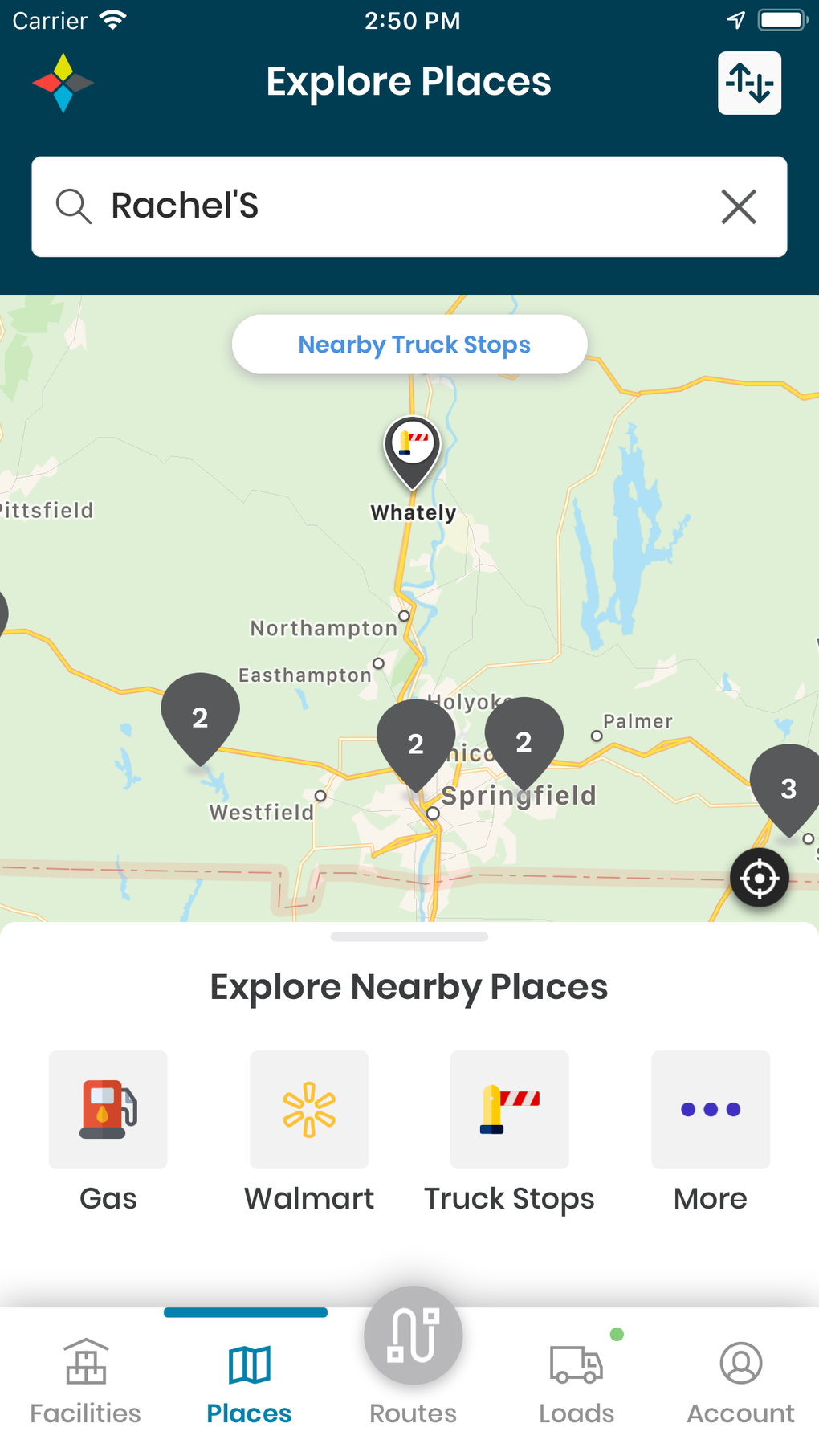The screenshot depicts an image captured on an iPhone at 2:50 pm, showing the full battery status and a strong WiFi connection. The carrier information is obscured. The displayed app is a map-based service that assists users in exploring various locations like Rachel's, possibly a truck stop, restaurant, or café, along with other key places such as gas stations, Walmart, truck stops, and additional facilities. The main section of the screen features a map with truck stops prominently marked: two near Westfield, two near Springfield, two between these locations, some near Northampton, and three on the right side of the map. The user appears to be specifically searching for Rachel's, although the nature of this location is unclear. The app interface also includes several options for the user to navigate, such as routes, loads, and accounts, with a green dot indicating a new notification in the "loads" section.